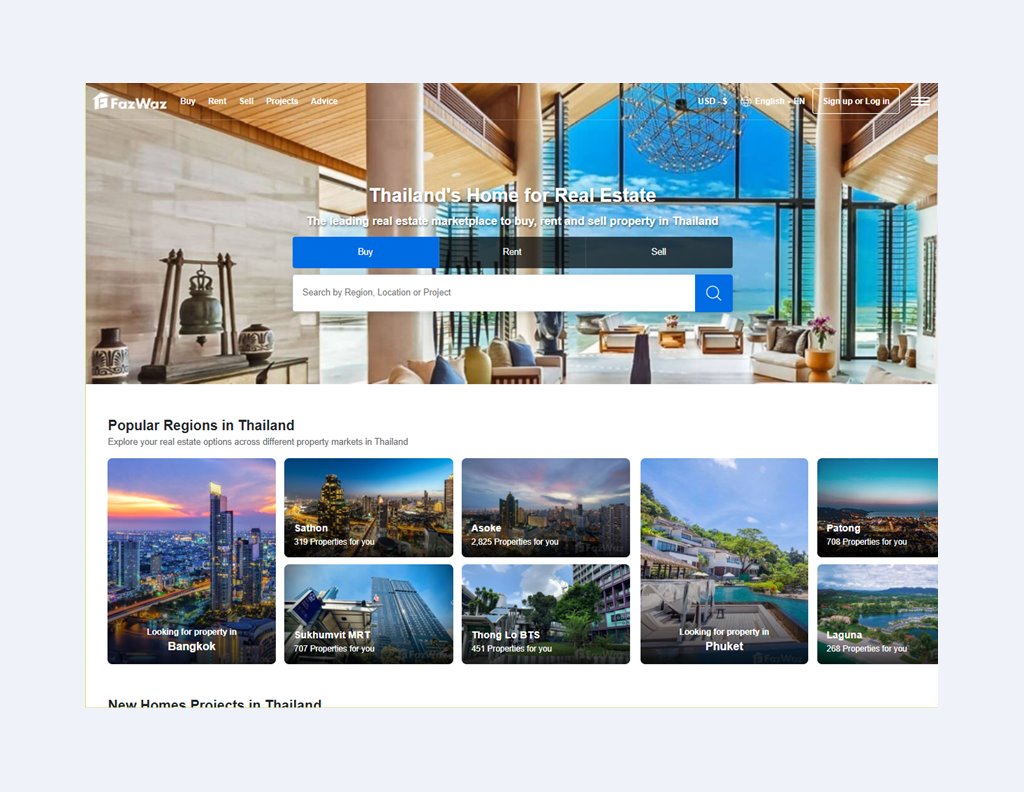The image features a modern, visually-appealing design with a light blue background. At the top left corner, there is a small white house icon next to the text "FazWaz," which is followed by options labeled "Buy," "Rent," and "Sell," along with two additional menu options. The central focus of the image is a stunning photograph of a beautifully decorated house with a large front window. Above this image, the text reads, "Thailand's Home for Real Estate," accompanied by a brief sentence in white font. Below, there are three prominently displayed buttons: a blue "Buy" button, and black buttons for "Rent" and "Sell." A white search bar with a blue magnifying glass icon sits below these buttons.

Further down, the image transitions to a white background featuring the header "Popular Regions in Thailand." Below this header are eight smaller images, each representing a different region: Bangkok, Sathorn, Sukhumvit, Asoke, Phrom Phong, Phuket, Patong, and Laguna, each with a beautiful, region-specific picture. At the very bottom, there is a partial view of a section labeled "New Home Projects in Thailand."